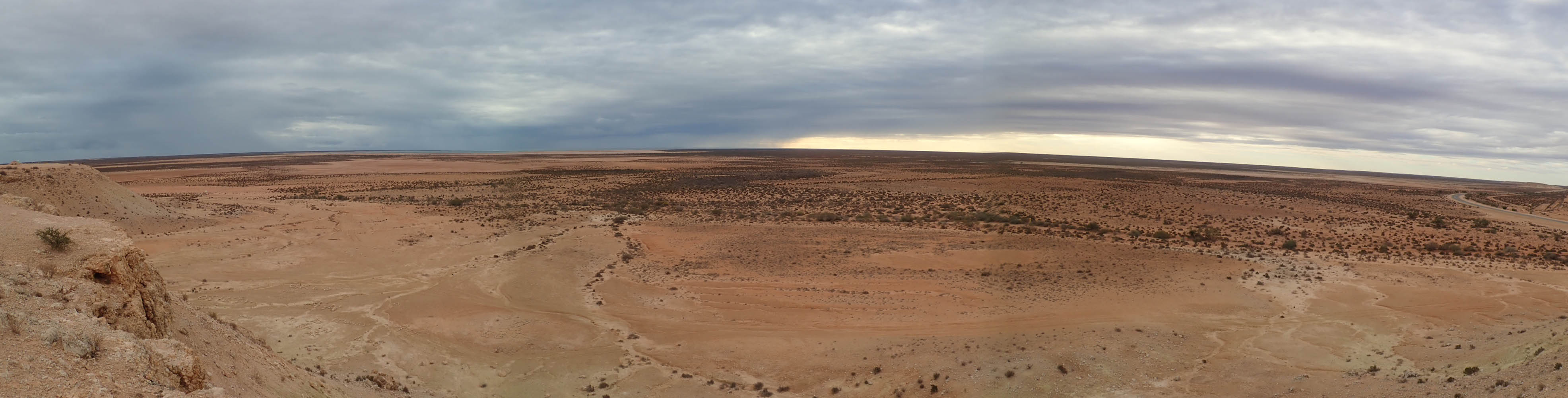This panoramic image captures a sprawling desert landscape with a wide view that encompasses several perspectives, stitched together seamlessly. The predominant colors are shades of orange, peach, and brown, characteristic of the sandy terrain. Sparse vegetation, including small shrubs and sagebrush, dots the windswept desert. On the left side of the image, a mountain range rises, with rock formations that match the sandy hue, interspersed with vegetation in certain lines along the slopes. The dark gray, cloudy sky looms overhead, suggesting an impending storm. The horizon, particularly on the right side, reveals a faint glimmer of light breaking through the clouds. This scene vividly conveys the vastness and rugged beauty of the desert environment.